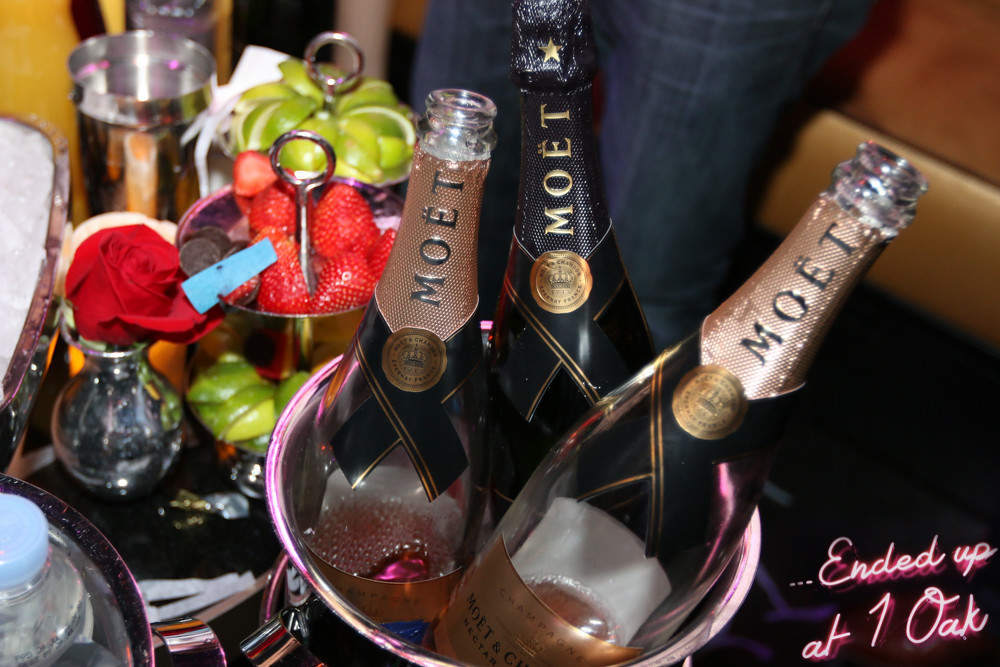The image depicts a silver bucket containing three mostly empty Moët & Chandon champagne bottles. The bottle on the left features a gold label with the brand name "Moet" prominently displayed. The center bottle also displays "Moet" but against a black label, while the bottle on the right has black letters on a gold label. A closer inspection reveals a bottle of water nestled among the champagne bottles in the bucket. The scene includes various details such as a bucket filled with strawberries and limes, adding a vibrant touch. A red rose is elegantly placed in a small, clear vase, sitting on a black table. In the background, a person, wearing dark pants, is pushing the lids behind the champagne bottles. Additionally, pink cursive text at the bottom right of the image against a black background reads, "ended up at 1 OAK," suggesting this scene is from a nightclub event.